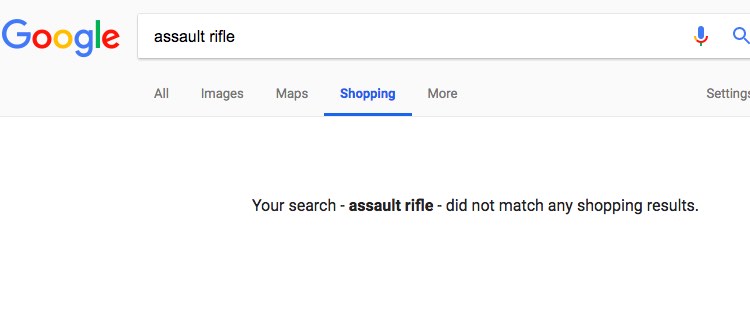The image is a screenshot displayed against a solid white background. In the upper left corner, the Google company name and logo are prominently featured with its characteristic blue, red, yellow, and green colors. To the right of the logo is a white search bar containing the bold black text "assault rifle." Adjacent to the search bar are the Google microphone icon and the blue magnifying glass icon. Below the search bar, there is a horizontal navigation bar. From left to right, the options listed are: "All," "Images," "Maps," "Shopping," with "Shopping" highlighted in blue and underlined. Following "Shopping" are "More" and "Settings." Beneath this bar, after a light gray horizontal line, there is another white space with the centered text: "Your search - assault rifle did not match any shopping results." The phrase "assault rifle" is in bold black text to emphasize the search query.